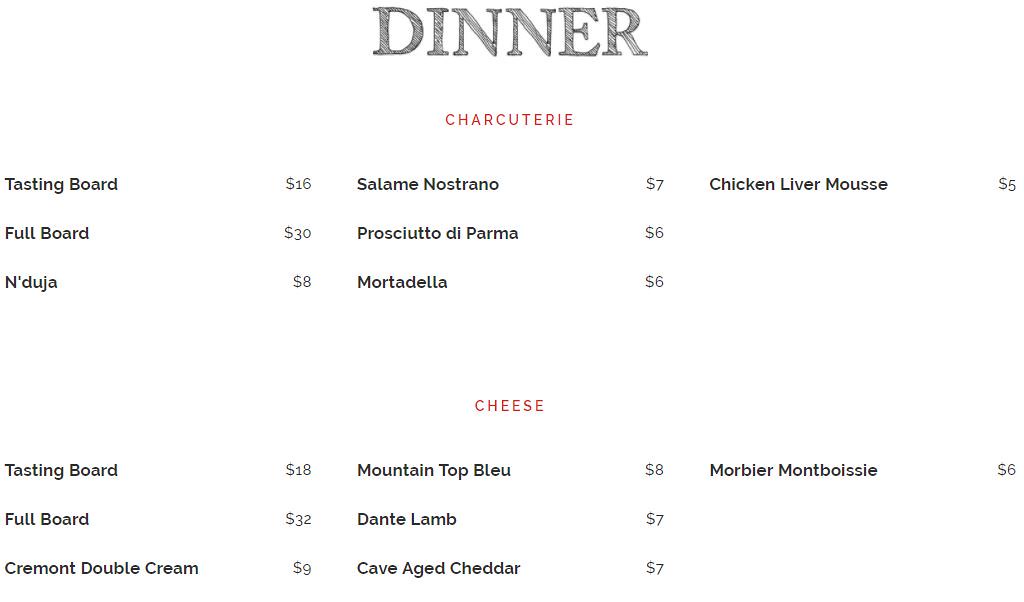The image is a part of a restaurant dinner menu with a white background. At the top center, in large black capital letters, it reads "DINNER." Below this, in red text, it says "CHARCUTERIE." The charcuterie section lists items in three columns: 
- Tasting Board for $16 
- Full Board for $30 
- Nduja for $8
- Salami Nostrano for $7 
- Prosciutto di Parma for $6 
- Mortadella for $6 
- Chicken Liver Mousse for $5.

Further down, also in red text, the menu features a "CHEESE" section, also organized in three columns: 
- Tasting Board for $18 
- Full Board for $32 
- Cremant Double Cream for $9 
- Mountaintop Blue for $8 
- Dante Lamb for $7 
- Cave Aged Cheddar for $7 
- Morbier Montblouse for $6. 

The layout is clean and organized into three columns, with the charcuterie and cheese sections distinctly separated by their red headings.